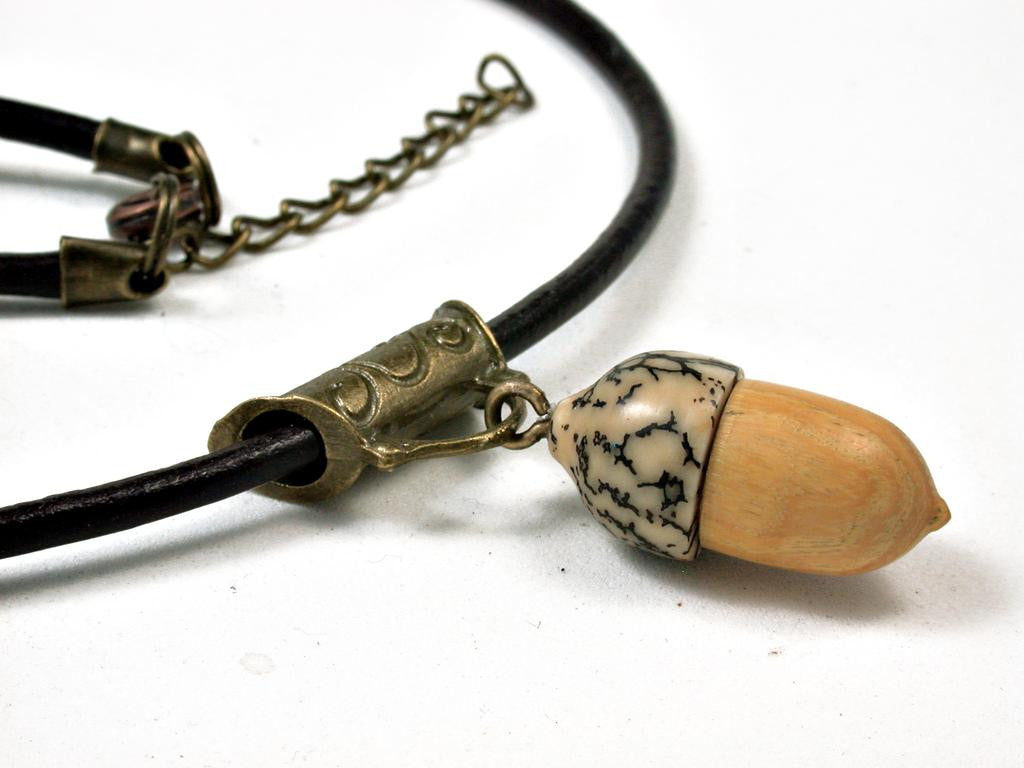The image is a close-up of a handmade jewelry piece, specifically a necklace featuring a detailed acorn pendant. The background is a very pale gray or white stone countertop, speckled with small bits. The necklace comprises a thick black cord that appears to loop and curve from the top center to the left side of the image, exiting and then re-entering from the upper left. At the forefront, attached to the black cord, is a gold-colored cylinder engraved with intricate designs. Hanging from the cylinder is an acorn pendant, with a cap made from a light brown stone or acrylic material marbled with black lines. The bottom part of the acorn is carved from a lighter colored wood. The black cord is capped with metallic pieces, likely gold or bronze, connected by a chain clasp that extends towards the top center of the image.